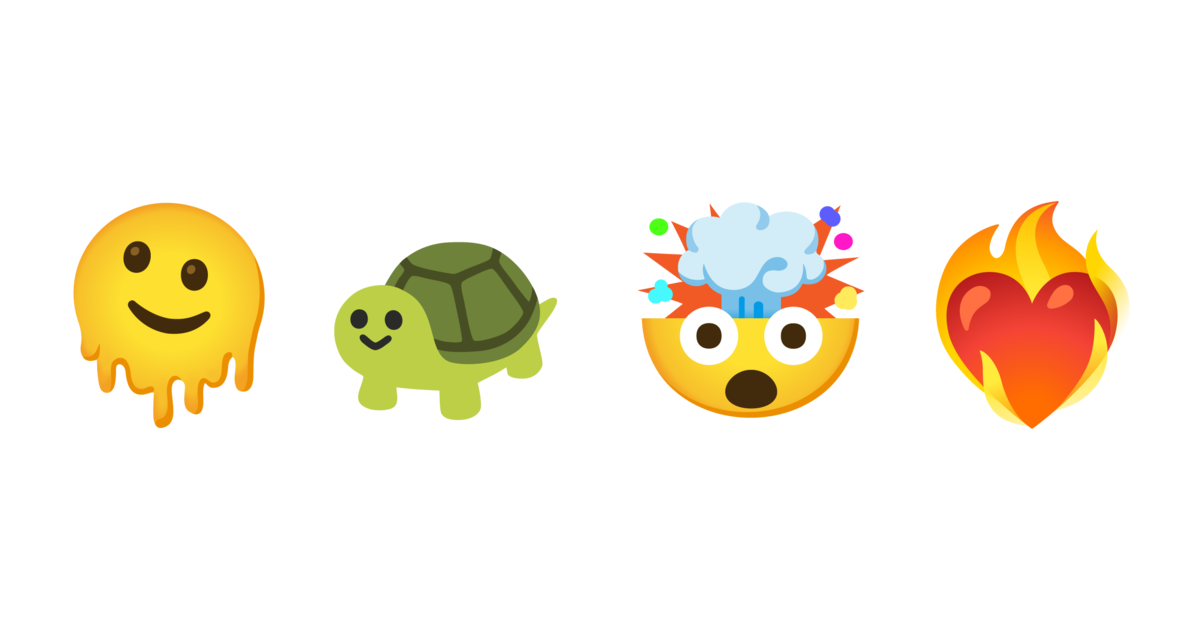Against a white background, four distinct emojis are arranged in a row. The leftmost emoji is a melting round-shaped yellow face with two black eyes and a smiley mouth that appears to be dripping at the bottom. To its right is a green turtle emoji, featuring a smiling face with two dark eyes and a V-shaped smile. The turtle's belly is a lighter shade of green, and its shell has a gray and black pattern. Next, there is an emoji of a shocked yellow face with wide-open black eyes encased in white circles and a large oval mouth; the top of its head is exploding. The rightmost emoji is a red heart engulfed in yellow flames, giving the appearance of a flaming heart.